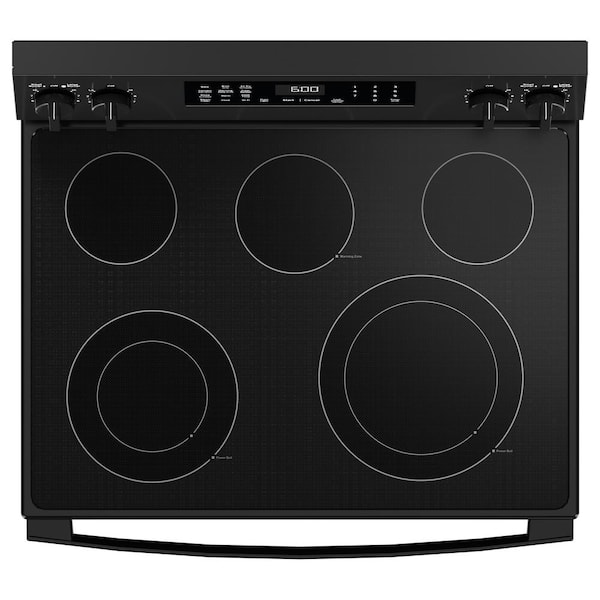The image displays a black matte-finish stovetop viewed from above. The stovetop features five burners: three of the same size arranged in the back row with slender white outlines, and two in the front row where the left burner is smaller than the right. The control interface includes four knobs—two on the left and two on the right—used to adjust the burners' temperature. Centrally located is an electrical clock set to 6:00, flanked by additional settings whose texts are not legible from this angle. Below the stovetop is a handle presumably for accessing the oven. The overall minimalist design employs only black and white colors for easy readability.